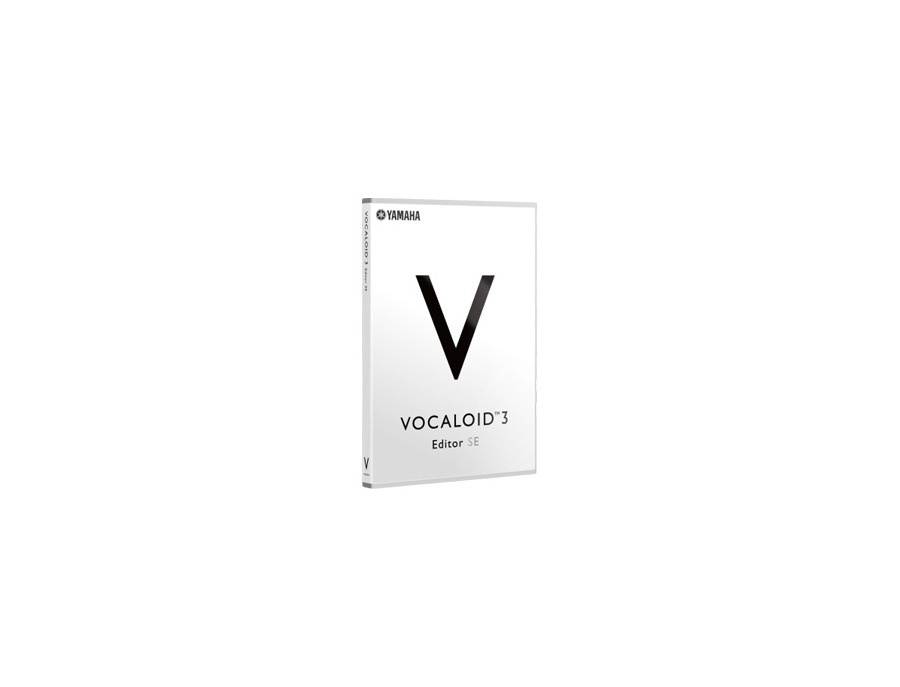The image depicts a small, vertically rectangular item that appears to be a software container, possibly resembling a thin book or a CD with a booklet. The cover features a gradient gray color scheme, with a lighter shade on top transitioning to a darker shade at the bottom. Dominating the cover is a large black "V" centered prominently. In the upper left-hand corner, a small circle contains a star along with the word "YAMAHA" in all caps. Below the large "V," the word "VOCALOID 3" is written in smaller black, all-caps letters, with the word "EDITOR" in an even smaller black font just beneath it, followed by the letters "SE" in gray. The spine, which is partially visible, has "VOCALOID" written vertically at the top and another capital "V" at the bottom. The overall background of the image is white, with gray shading adding to the details.